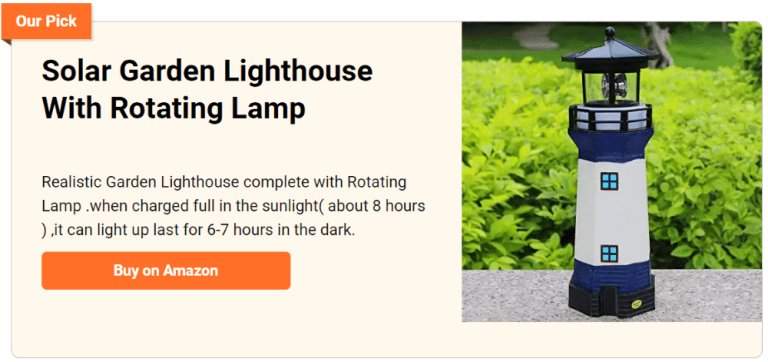On a beige background, the right side features a colorful image of a small solar-powered lighthouse-shaped light, styled in white and navy blue. The lighthouse is positioned on a concrete surface, with a vibrant green bush in the background providing a natural contrast. In the upper left corner of the image, a small orange rectangle with white text reads "RPIC." Dominating the beige background is large black text that states, "Solar Garden Lighthouse with Rotating Lamp." Beneath this, in smaller text, a detailed description reads: "Realistic garden lighthouse complete with rotating lamp. When fully charged in sunlight (approximately eight hours), it can illuminate and last for six to seven hours in the dark." Below this description, an orange button with white text in the center invites viewers to "Buy on Amazon."